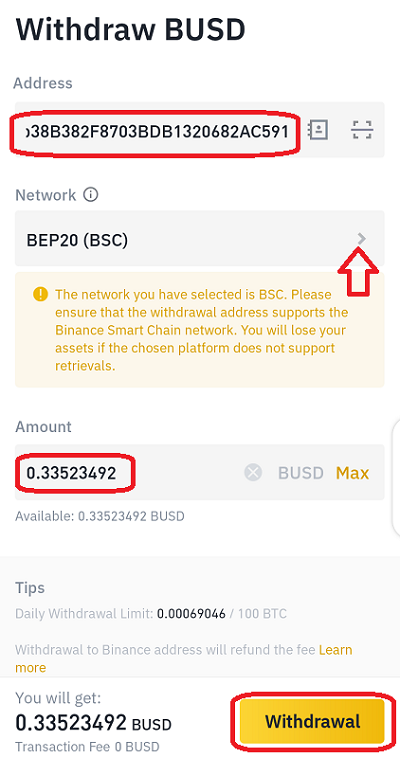Here's a detailed, cleaned-up caption for the image describing the web page for withdrawing BUSD:

---

The image captures a web page interface for withdrawing BUSD, structured with sections of text on a white background. At the top, the heading "Withdraw BUSD" is displayed in black. Below it, the word "Address" appears in gray, followed by a gray box containing the sequence of numbers and letters of the address. Underneath, the term "Network" is presented in gray, with a gray bar indicating "BEP20 (BSC)" in a ribbon. 

On a pink background, golden text beginning with an exclamation point inside a circle warns: "The network you have selected is BSC. Please ensure that the withdrawal address supports the Binance Smart Chain Network. You will lose your assets if the chosen platform does not support retrievals." A red arrow points upward to the circled address, emphasizing its importance.

Moving down, the term "Amount" is shown in gray, with the amount "0.33523492 BUSD" displayed in a gray ribbon. Adjacent to it, "Max" is written in gold. Below, "Available 0.33523492 BUSD" is noted in gray. 

A light gray box labeled "Tips" provides additional information. This includes, in gray text: "Daily withdrawal limit: 0.00069046/100 BTC" and "Withdrawals to Binance address will refund the fee." The phrase "Learn more" is highlighted in gold.

At the very bottom, it states "You will get 0.33523492 BUSD" followed by "Transaction fee: 0 BUSD." To the right, a prominent gold button with the text "Withdraw" in black is circled in red, indicating where to click to complete the withdrawal.

---